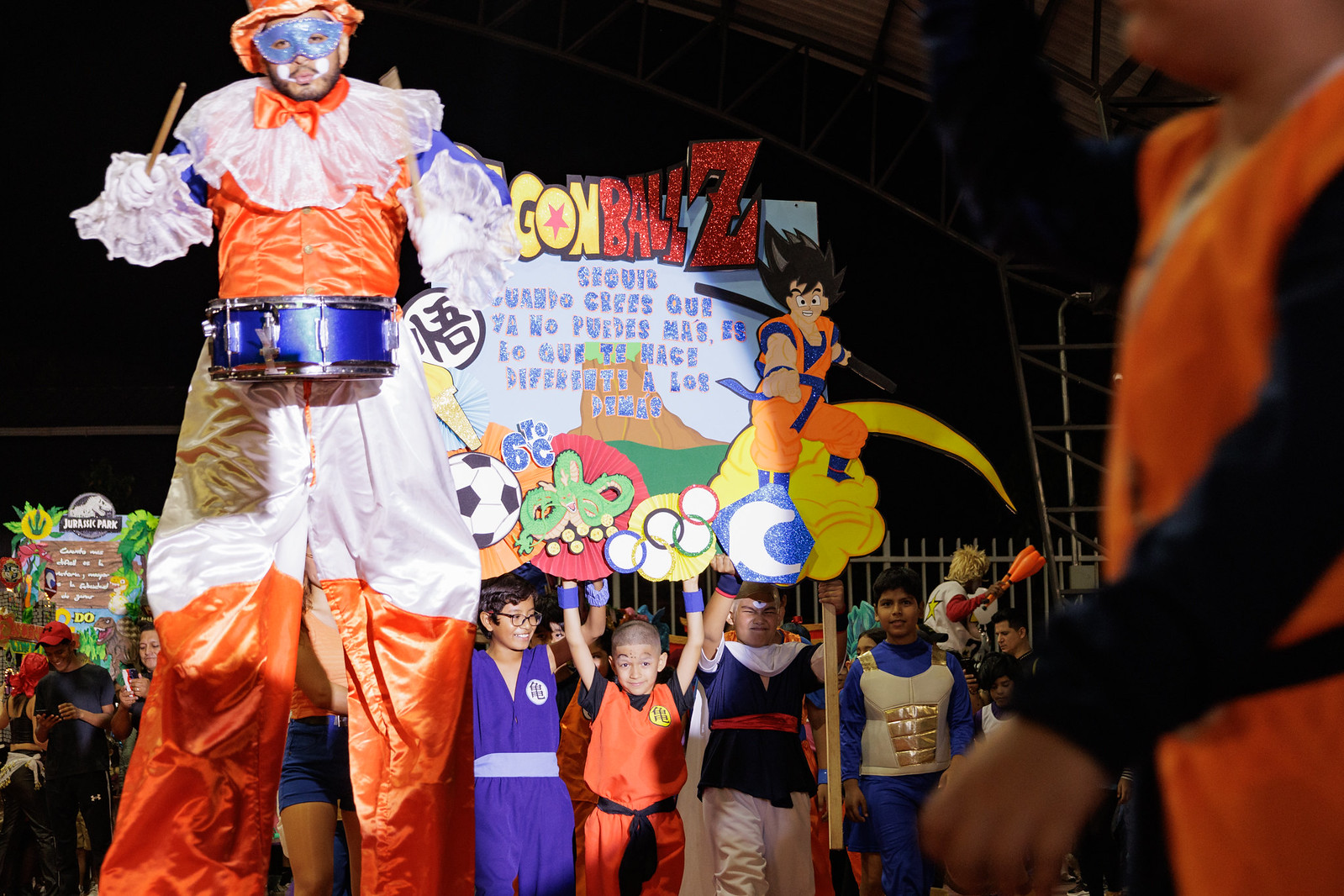The image captures a lively celebration of Dragon Ball Z, possibly a circus or parade event. In the foreground, a tall man on stilts commands attention with his striking attire: voluminous pants that fade from white at the top to orange at the bottom, an orange shirt with blue sleeves, and white sheer frills around his wrists and neck. His face is partially obscured by a blue mask covering his eyes, and he's topped with an orange bucket hat. The man is playing a blue drum, held with brown drumsticks in both hands. 

Behind him, a sign prominently displays "Dragon Ball Z" followed by several words in Spanish written in blue. Scattered around are numerous participants, many dressed in cosplay costumes from Dragon Ball Z, including martial arts uniforms in shades of blue and orange. The festive atmosphere is amplified by children in various costumes, some reminiscent of anime characters, and vibrant decor referencing elements like soccer and the Olympic rings. Despite the man's colorful garb and the joyous scene, his expression seems incongruous, appearing more disgusted than delighted.